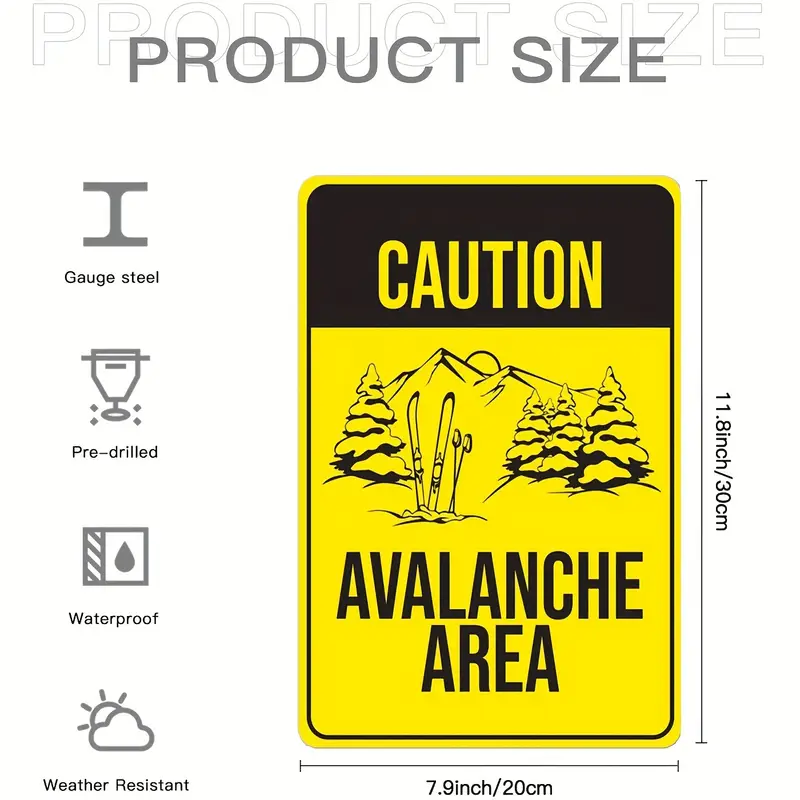The image depicts a rectangular caution sign designed for avalanche areas, typically used at ski resorts. The top of the image features a gray banner with the text "Product Size," indicating the sign's dimensions: 7.9 inches by 11.8 inches (20 cm by 30 cm). The sign itself is prominently yellow with black text and graphics. At the top of the sign, the word "CAUTION" is highlighted in yellow on a black background stripe. Below this, the main body of the sign displays an illustration of a mountain with two skis and poles protruding from the snow, suggesting a dire avalanche scenario. Below the image, the words "AVALANCHE AREA" are boldly printed in black. The left side of the image features several icons illustrating the sign's features: gauge steel material, pre-drilled for easy mounting, waterproof, and weather-resistant, each accompanied by corresponding graphics such as a drill, water drop, and cloud with the sun. The overall presentation suggests this is a product listing from a website specializing in safety signage for ski resorts.